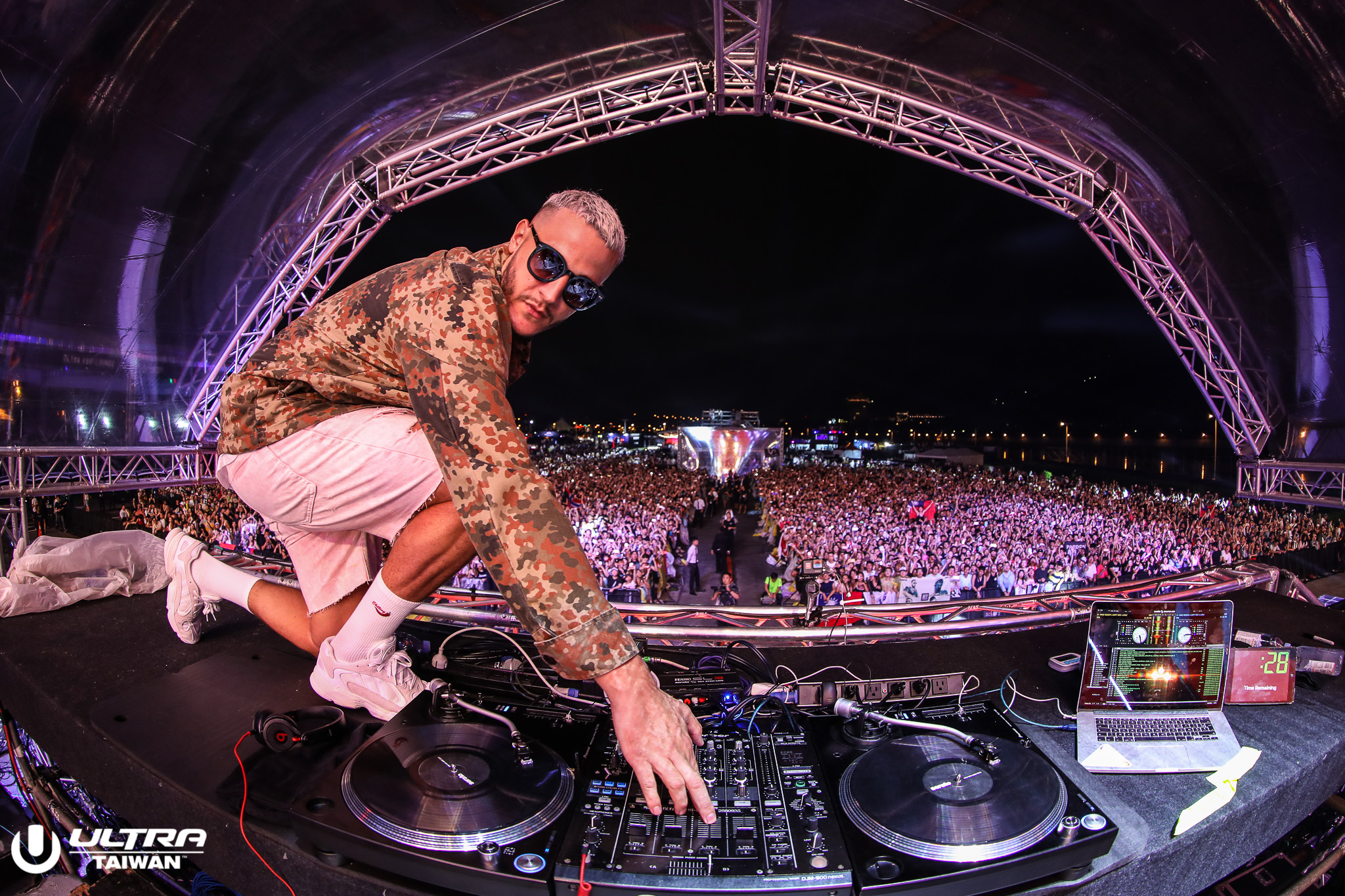In this dynamic photograph captured through a fisheye lens, a DJ is energetically performing on a large outdoor stage at night. He is dressed in a long-sleeved camouflage-patterned shirt, khaki shorts, white socks, white shoes, and sports sunglasses along with short, dyed blonde hair and a dark goatee. The DJ is kneeling on the table, deeply focused as he manipulates his mixing panel and dual turntable setup. To his right, a thin silver laptop displays a music interface complete with a sound graph and timer. Below the DJ, the crowd extends endlessly from the edge of the stage into the distance, split by a central aisle with lights illuminating the vast audience. The bottom left corner of the picture bears a white "Ultrataiwan" watermark, suggesting the event's location in Taiwan. The stage is large and illuminated, creating a mesmerizing atmosphere where music and energy unite.